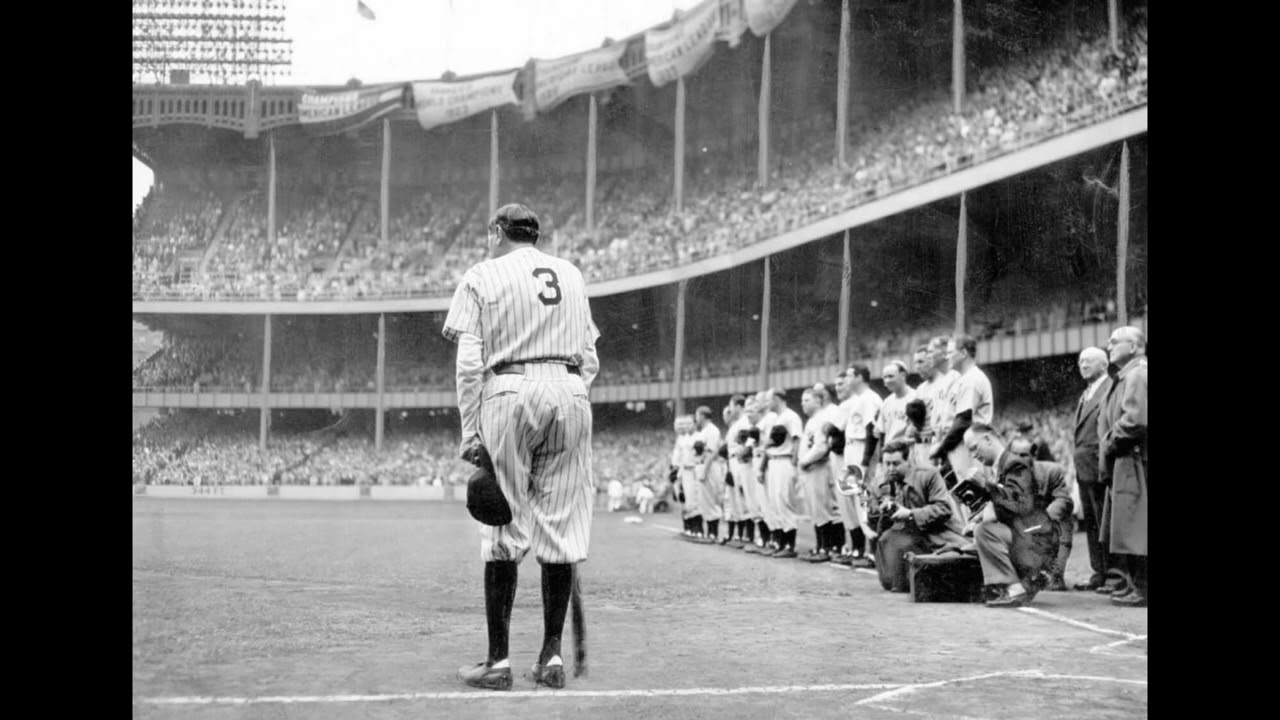The black-and-white photograph captures a historic moment at a packed baseball stadium. The main subject of the image is the legendary Babe Ruth, distinguished by his signature number three on the back of his old-timey pinstriped Yankees uniform. Ruth stands near home plate, holding a bat in his right hand with its top resting on the ground, while his other hand, loosely by his left knee, holds his black baseball cap. He is surrounded by a line of fellow baseball players who stand solemnly with their hats over their hearts, suggesting the playing of the National Anthem. The stadium is filled to the brim with spectators, stretching across three tiers, with details of banners flying from the roof and metal cages holding lights illuminating the scene. To Ruth's right, several photographers kneel on the ground to capture the moment, along with two men in suits and overcoats. The scene is vivid, capturing both the grandeur of the moment and the reverence of the occasion.